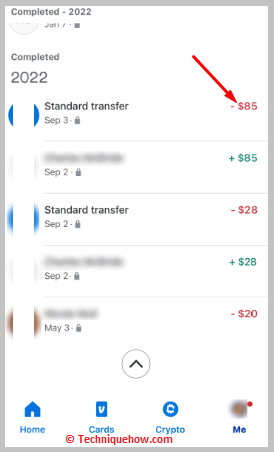This is a detailed screenshot from techniquehow.com showcasing various standard transfer transactions. 

At the top, the text "Completed 2022" is prominently displayed, repeated below in a larger font size. The first entry documents a standard transfer resulting in a debit of £85, highlighted in red font with a red arrow icon pointing to this amount. The subsequent transaction is blurred for privacy, with the only visible detail being a credit of $85 in green font located in a different column.

Further down, another standard transfer is listed, showing a debit of $28 in red font in the far column, dated 2nd of September. Similar to the earlier redacted entry, another transaction on the 2nd of September is blurred but indicates a credit of $28 highlighted in green font. Lastly, there is a redacted entry from May 2nd, depicting a debit of $20 in red font.

All these transactions are timestamped and fall under the same date format, providing a comprehensive view of the financial activities and their respective amounts, categorized by color codes to distinguish between debits in red and credits in green.